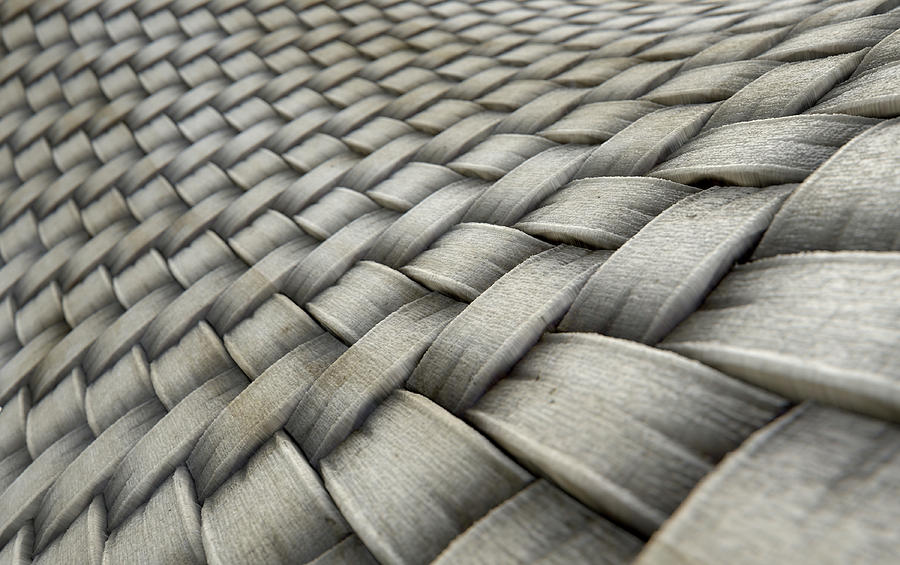This image is a highly detailed, zoomed-in shot of woven fabric strips, which might also resemble the weaves of a basket. The thick, grayish-white fabric strips, some of which are stained with a bit of brown, are intricately woven over and under each other in a uniform pattern that stretches across the entire picture. The weave exhibits a rough texture, and part of the fabric is angled, offering a closer and more detailed foreground view while zooming out gradually to reveal the full pattern. This close-up depiction showcases the meticulous weaving process, where each strand interlocks to form a strong, cohesive whole, suggesting it could have been taken from a factory setting where such weaves are created. The image is devoid of any text or additional objects, focusing solely on the texture and pattern of the weave.